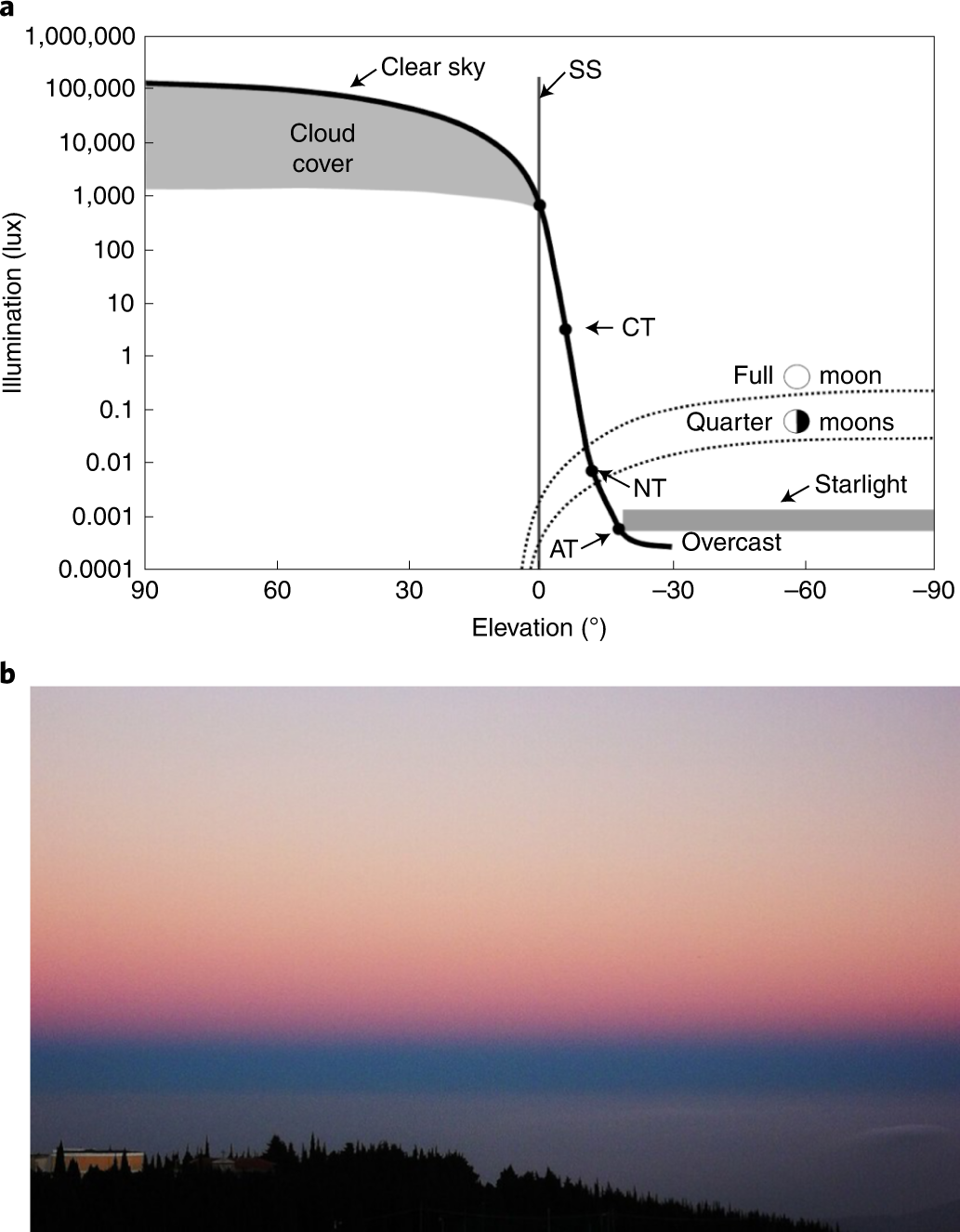This image consists of two parts: a detailed diagram and a photograph. The diagram, labeled A, is a line graph showing illumination measured in lux on the y-axis, ranging from 0.0001 to 1 million, and elevation measured in degrees on the x-axis, spanning from 90 to -90. The graph features a prominent dark line that steeply descends at zero elevation, marked SS, indicating a significant drop in illumination. Dotted lines for full and quarter moons provide additional reference points, and the graph highlights the effects of cloud cover, starlight, and overcast conditions on illumination levels.

Below the diagram, the image contains a low-quality photograph capturing a sky at either sunrise or sunset, displaying a gradient of colors from pale pink to dark blue. The sky is cluttered with clouds, resulting in limited visibility. Situated at the lower left corner of the photo is a yellow building, possibly an observatory, surrounded by an extensive tree line comprising pine trees stretching from the right side of the building to the lower right section of the image.